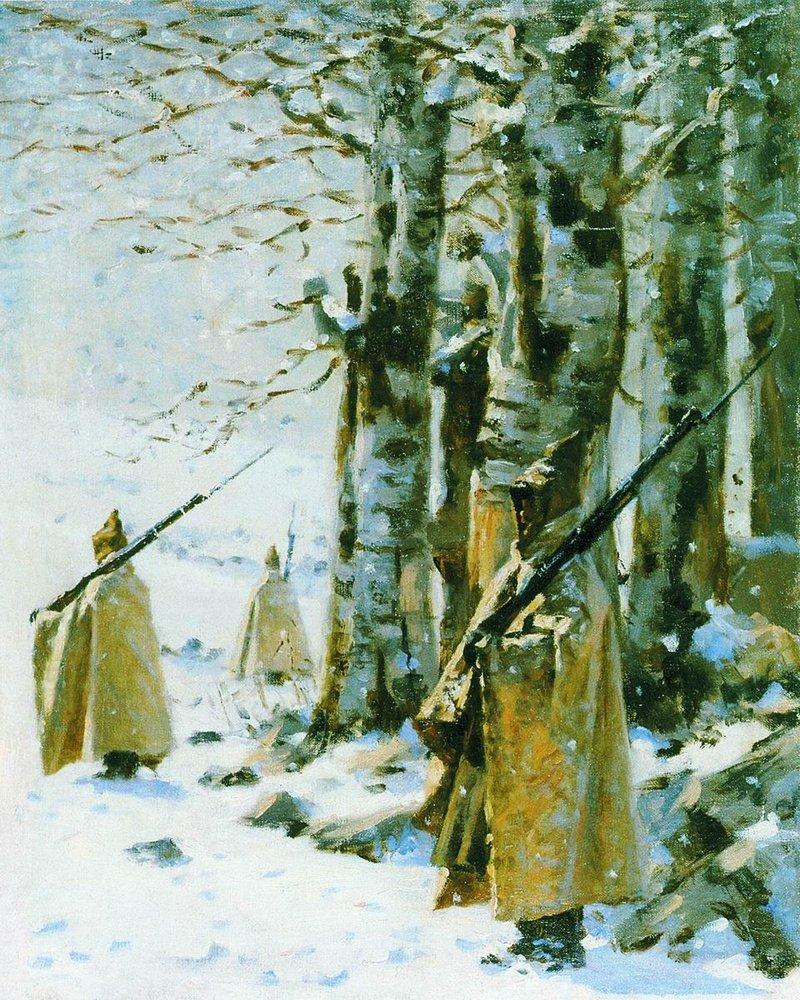The artwork is a detailed oil painting rendered in an impressionist style, depicting a trio of soldiers in a harsh winter landscape, possibly dating back to the 19th century or the Civil War era. The scene unfolds outdoors during the day, covered in a blanket of white snow. Each soldier wears a yellow or tan poncho with a pointed hood, designed to shield them from the cold and elements. Their dark pants and boots contrast sharply with the snow-covered ground. All three soldiers grasp long, old-style rifles with bayonets, draped over their shoulders with their left hands. 

The composition positions one soldier at the forefront, partially turned sideways so his face is faintly visible beneath the hood. The other two soldiers stand behind with their backs turned towards the viewer. Towering, thick-trunked, leafless trees fill the background, their black and white bark starkly standing out against the wintry whiteness. The setting is devoid of any text, focusing entirely on the scene's atmospheric and historical essence.